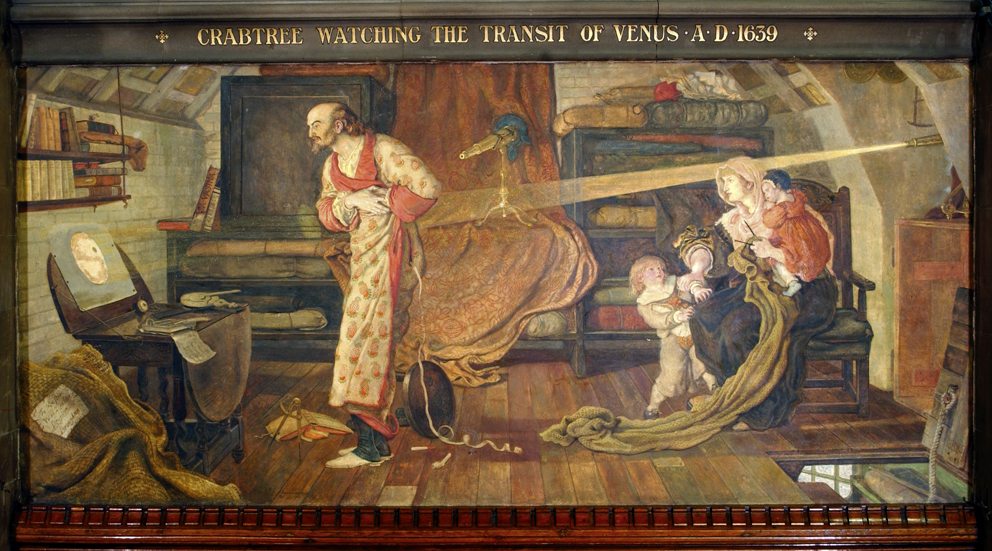A very detailed and atmospheric painting, titled "Crabtree Watching the Transit of Venus, A.D. 1639" in gold letters at the top, depicts a historical scene with intricate details and a sense of scientific observation. The painting appears old, rendered in an older style possibly from the 1700s. The central figure is a balding man wearing a robe with a floral pattern and pink trim around the neck and arms. He is engrossed in observing a piece of paper on a folding table, which reflects an image projected through a telescope across the room, likely capturing the transit of Venus across the sun. 

The room is cluttered with scientific equipment, including another telescope on a table, shelves with books, rolled-up parchment, and fabric. To the right, a woman sits on a wooden chair holding an infant, with a toddler beside her. The woman appears to be keeping the children at bay while watching the man's observations with a sense of astonishment. The beams of light from the telescope create a dramatic focus on the man's work. The woman's chair and the surrounding furniture give the room a lived-in, yet scholarly atmosphere, reflecting the man's deep involvement in scientific research.